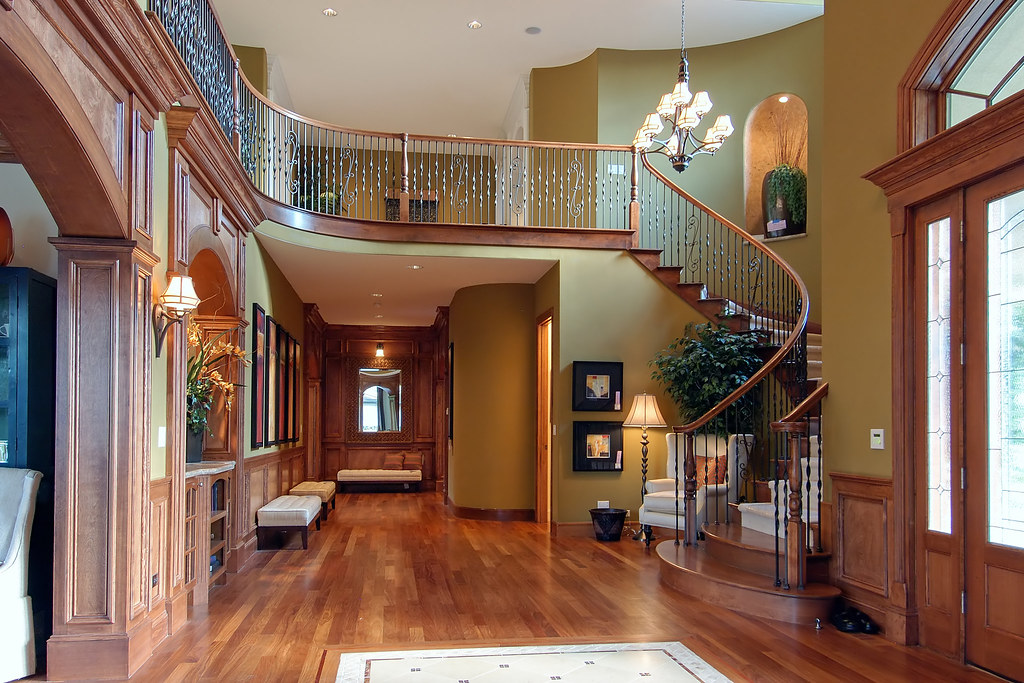The image captures the elegant foyer of a beautifully designed house. To the right side of the image stands a set of double brown wooden doors adorned with glass windows on the top two-thirds, allowing ample light to pour in. Adjacent to these doors, starting towards the middle of the image, a gracefully curved staircase ascends towards the left. The stairs are complemented by intricate railings featuring brown wood on top and decorative bars. A chandelier hangs prominently above the top steps of the staircase. Just beneath the curve of the staircase is a cozy nook with a white sofa chair accented by a brown cushion, accompanied by a plant, a reading lamp, and two stacked paintings. The center floor area consists of a charming wooden tile floor, blending medium and light brown shades, with segments of a white area rug featuring a subtle pattern. The foyer opens to the left through an arched entranceway that reveals part of a white chair in another room. Above the center of the image, spanning across the scene, is a high white ceiling embedded with spotlights. The walls appear to be painted green, further enriching the space with color, while white edges line various areas, adding refined details to the room's aesthetic.